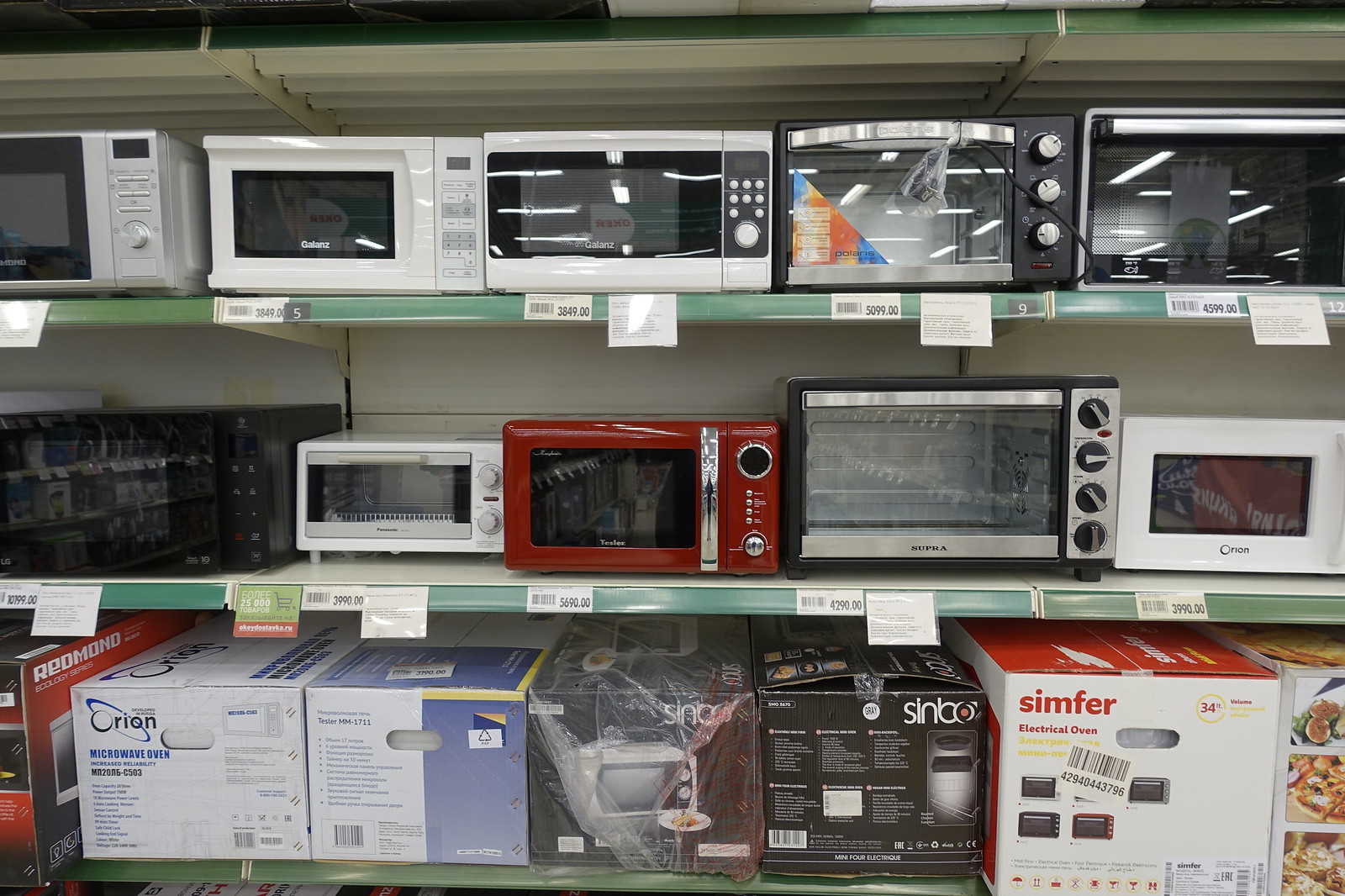The image depicts three shelves in a large retail store, possibly a Walmart, displaying a variety of microwaves, toaster ovens, and electrical ovens. The shelves are white with dark green fronts that display prices and informational cards.

On the top shelf, there are five appliances, starting from the left: a silver microwave, followed by a white microwave, another white microwave with gray details, a black microwave with silver handles, and then what appears to be an electrical oven. The appliances vary in shades and features.

The middle shelf holds five more appliances, starting from the left: a black microwave, a small white microwave, a retro red toaster oven, a medium-sized white toaster oven or electrical oven, and another small microwave.

The bottom shelf contains seven boxed appliances, with brands and models somewhat obscured by plastic wrapping and partial obstruction. Among these boxes are a Redmond appliance, a Ryan microwave oven, and a Simfer electrical oven. The specific details of the other boxes are unclear due to obstructed views.

Overall, the shelves are neatly organized, showcasing a wide range of kitchen appliances in various sizes, colors, and designs.